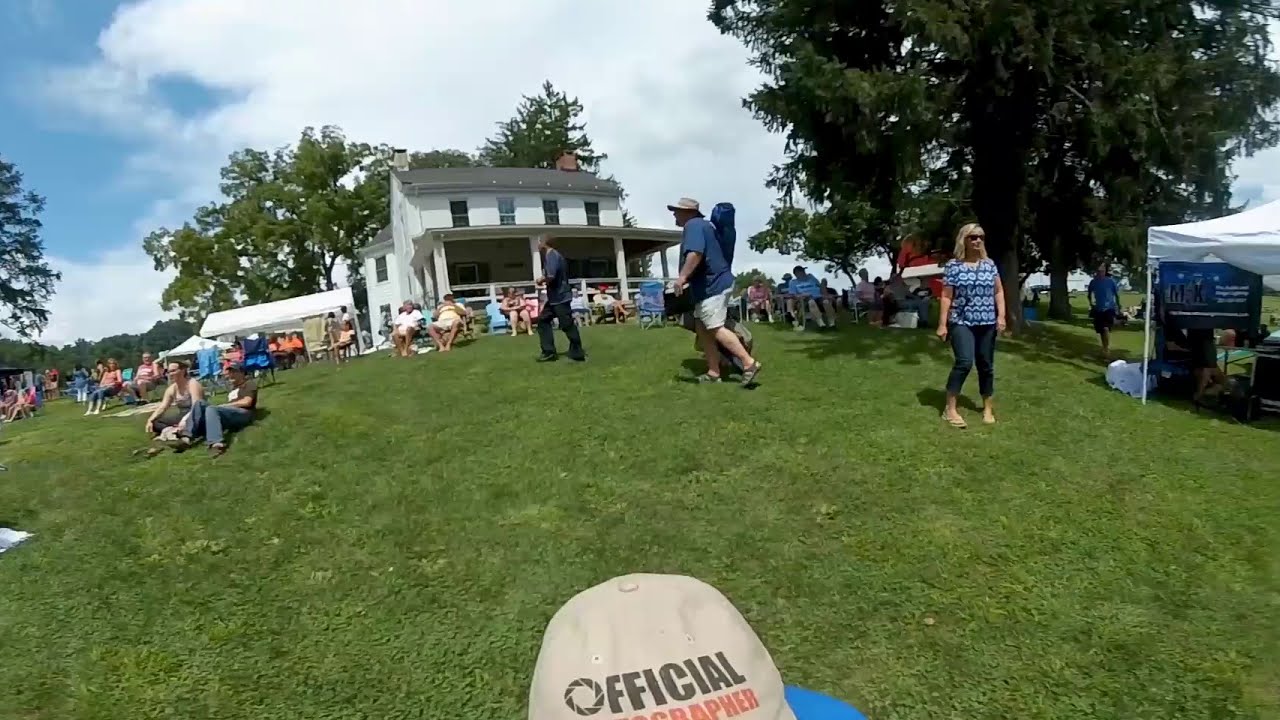This detailed image captures a lively outdoor event at Jim Dietrich Park in Pennsylvania, in front of a preserved, two-story, white plantation-style house with a large porch. The expansive grassy area is dotted with numerous attendees, some seated on lawn chairs and blankets, while others meander about. The scene reveals a sunny day with scattered clouds, dominated by a few towering green trees. On the left side, two people sit on the grass, one nearly lying down, while the majority, seated facing left at an angle, suggests a gathering focused on live music or a similar attraction. The participants appear prepared with various personal items like sunscreen, and chairs to enjoy the event. Centrally, a man in a blue shirt and a sun hat walks towards the left, possibly holding an instrument case, alongside another individual. On the right side, under a white-covered tent adorned with blue advertising letters "MX" and some unreadable writing, a lady in a t-shirt, pants, and sunglasses stands. The bottom center of the image features the top of a baseball cap with the words "Official Photographer" partly visible, hinting at the role of the individual taking the photograph.